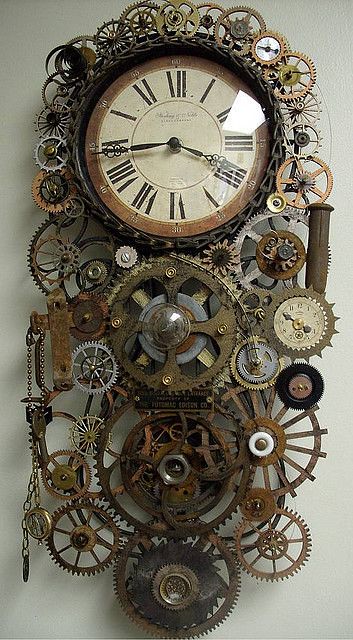The image showcases a steampunk-inspired clock hanging on a plain white wall, captured from a first-person POV. The clock is ornate, featuring a mix of rusted steel, gold, and black cogs and wheels arranged intricately around and beneath the main clock face. The numbers on the face are Roman numerals, with black clock hands indicating the time as approximately 3:44. The main clock face is enclosed in a black circular frame and covered by a reflective glass dome. Surrounding the face, and extending downward in a rectangular formation, are numerous decorative cogs and wheels, some of which have dangling pocket watches and keys, adding to the intricate and mechanical aesthetic.